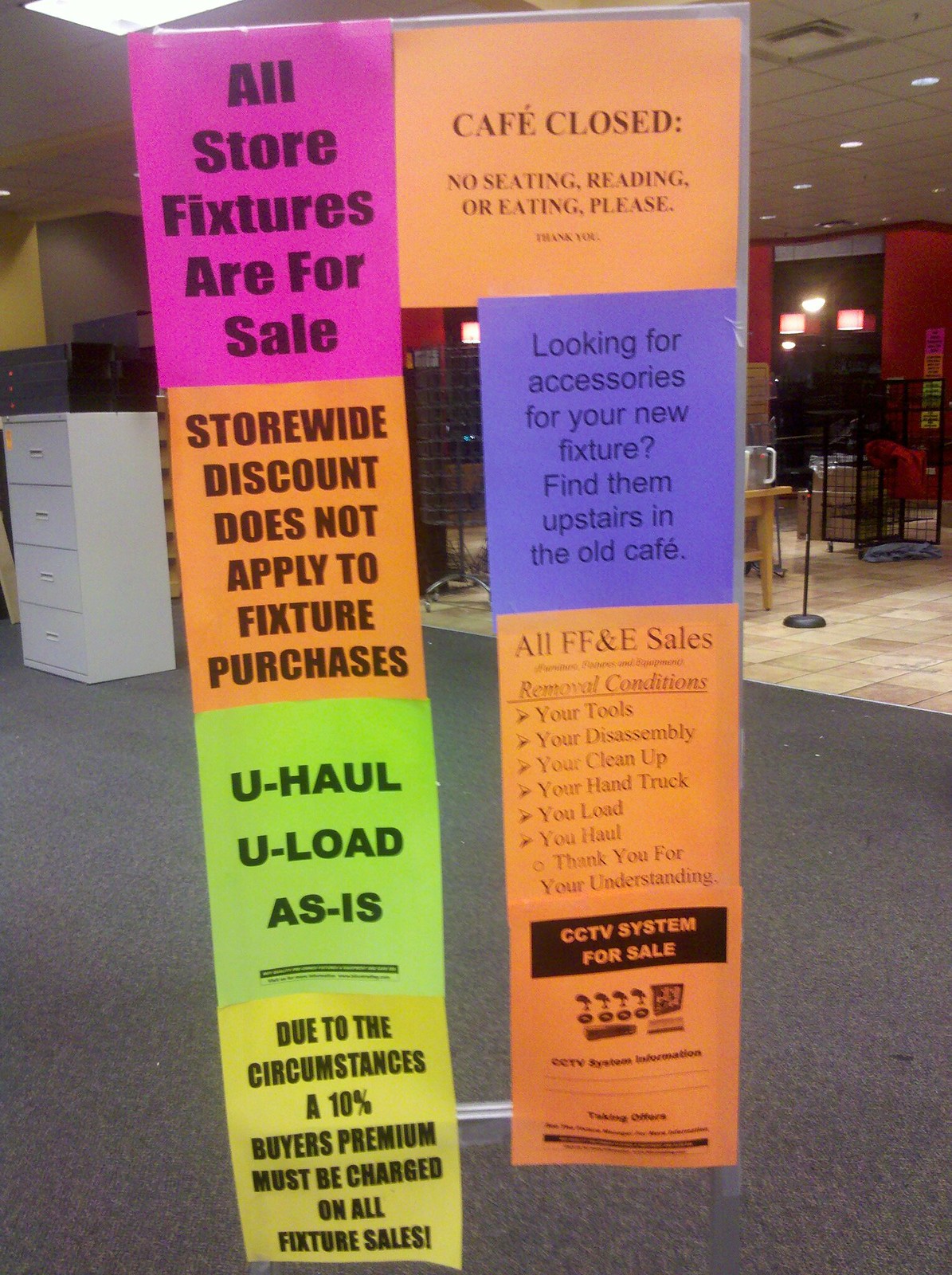A collection of eight vibrant sheets of colored paper, featuring large black text, are taped to the entrance of a building, likely a store. These signs, possibly affixed to a glass door, are primarily promotional and informational. The top-left sign announces, "All store fixtures are for sale." Adjacent to this, on the top-right, is a notice, "Cafe closed. No seating, reading, or eating, please." Additionally, there's a reminder that "Storewide discount does not apply to fixture purchases." Another sign guides customers, "Looking for accessories for your new fixture? Find them upstairs in the old cafe," which is now closed. Among other notices, one sign reads, "U-Haul. U-Load. As is," and another details conditions for sales and removals, emphasizing, "All FF&E sales: Your tools, your disassembly, you clean up, your hand truck." The text across these signs highlights logistical details about the sale and the status of the cafe, reflecting a business in transition. In the background, the store’s interior features a mix of brown and white tiled flooring transitioning into gray carpet, a cabinet with multiple drawers, and some scattered furniture pieces.